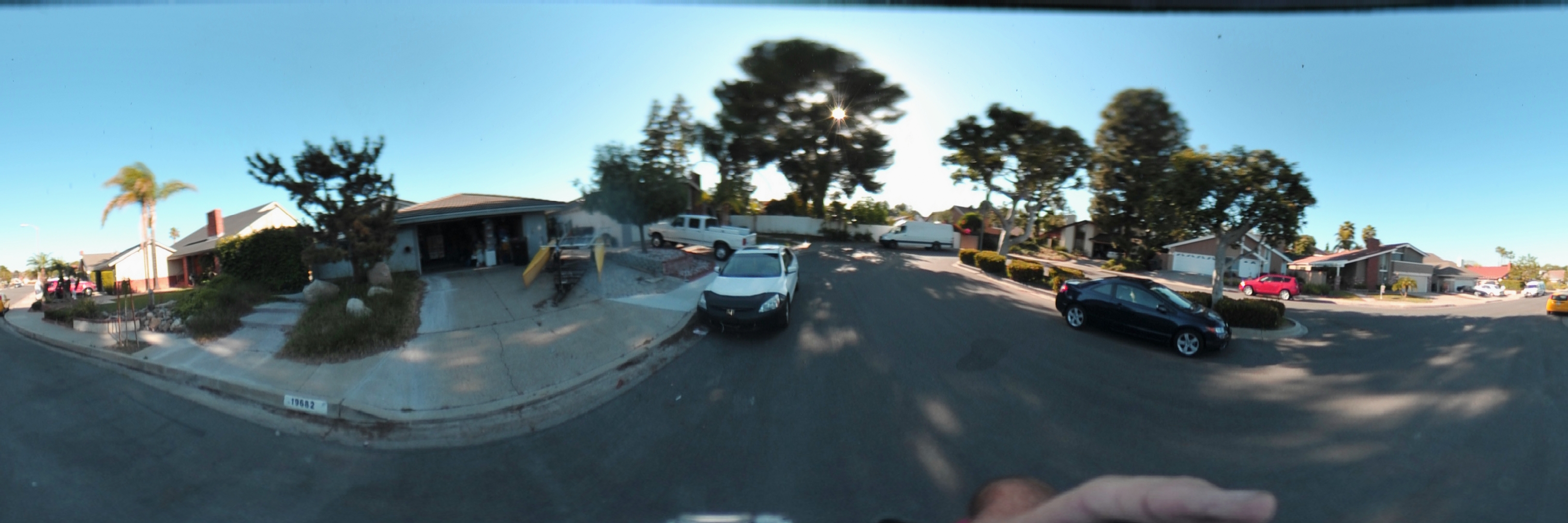A panoramic outdoor image of a picturesque neighborhood taken with a fisheye lens capturing a wide field of view. The clear blue sky dominates the background, with the sun positioned near the center on the horizon. The scene features a variety of trees, including tall, thin ones, plush or bulbous-topped trees, and even a small tropical palm tree. On the left side of the image, there are at least three houses: a prominent white one, a possibly off-white or slightly darker one, and another house painted in a darker hue. The right side showcases a gray garage with two large white doors and an adjacent darker-colored house, along with other less discernible structures. A visible street curves to the left with a curb line, while another road extends to the right. Various vehicles populate the neighborhood, including a small black car in motion, a stationary red car, a white car, and a white pickup truck parked nearby.